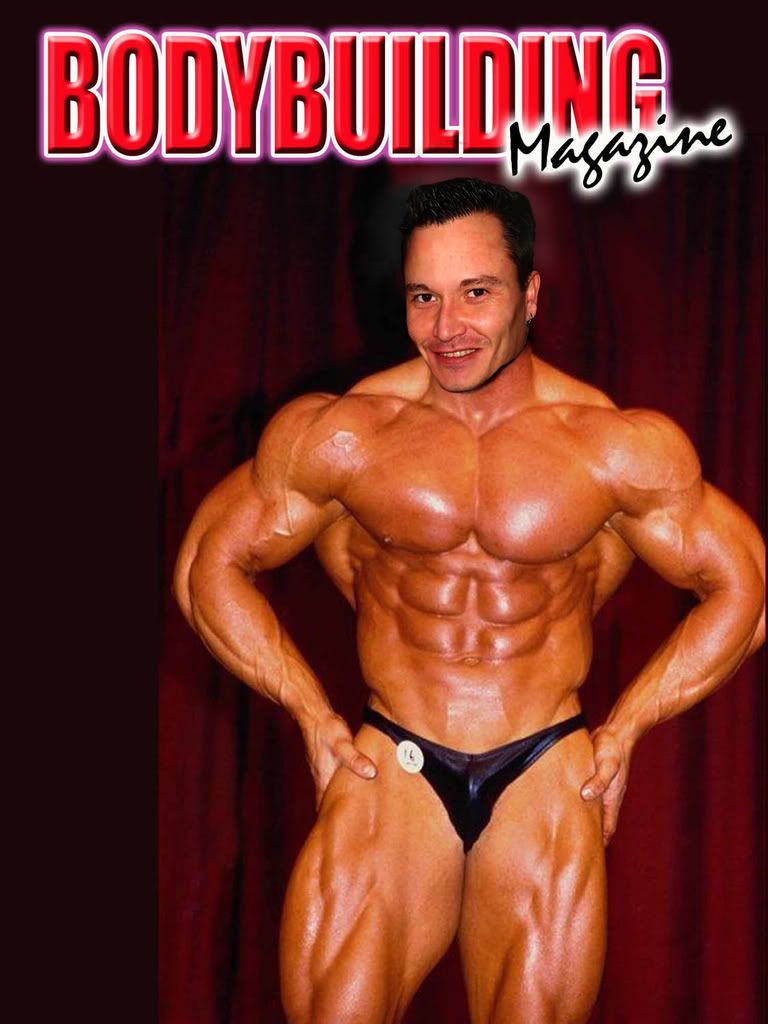The magazine cover features a manipulated photograph of a muscular man, prominently showcased from the knees up. The most striking element is his unnaturally proportioned, glistening, veiny musculature, garbed only in a tight, black Speedo adorned with a small circular tag marked with the number 16. Notably, his head appears digitally edited and mismatched in skin tone compared to the rest of his body, implying a heavy post-edit or Photoshop alteration. He has short hair and is smiling, engaging directly with the camera. His pose exudes confidence, with his hands firmly on his hips, showcasing his broad chest and defined arms.

The man stands against a dark red curtain backdrop, under the prominently displayed title "Bodybuilding Magazine". The word "Bodybuilding" is emblazoned across the top in bold, red capital letters outlined in black and white, while "Magazine" is elegantly inscribed beneath in black cursive font with a white outline. From his position in the center, semi-transparent white watermarks overlay the image: “photobucket” spans his chest, accompanied by a logo symbol, and a banner below it reads “protect more of your memories for less.”